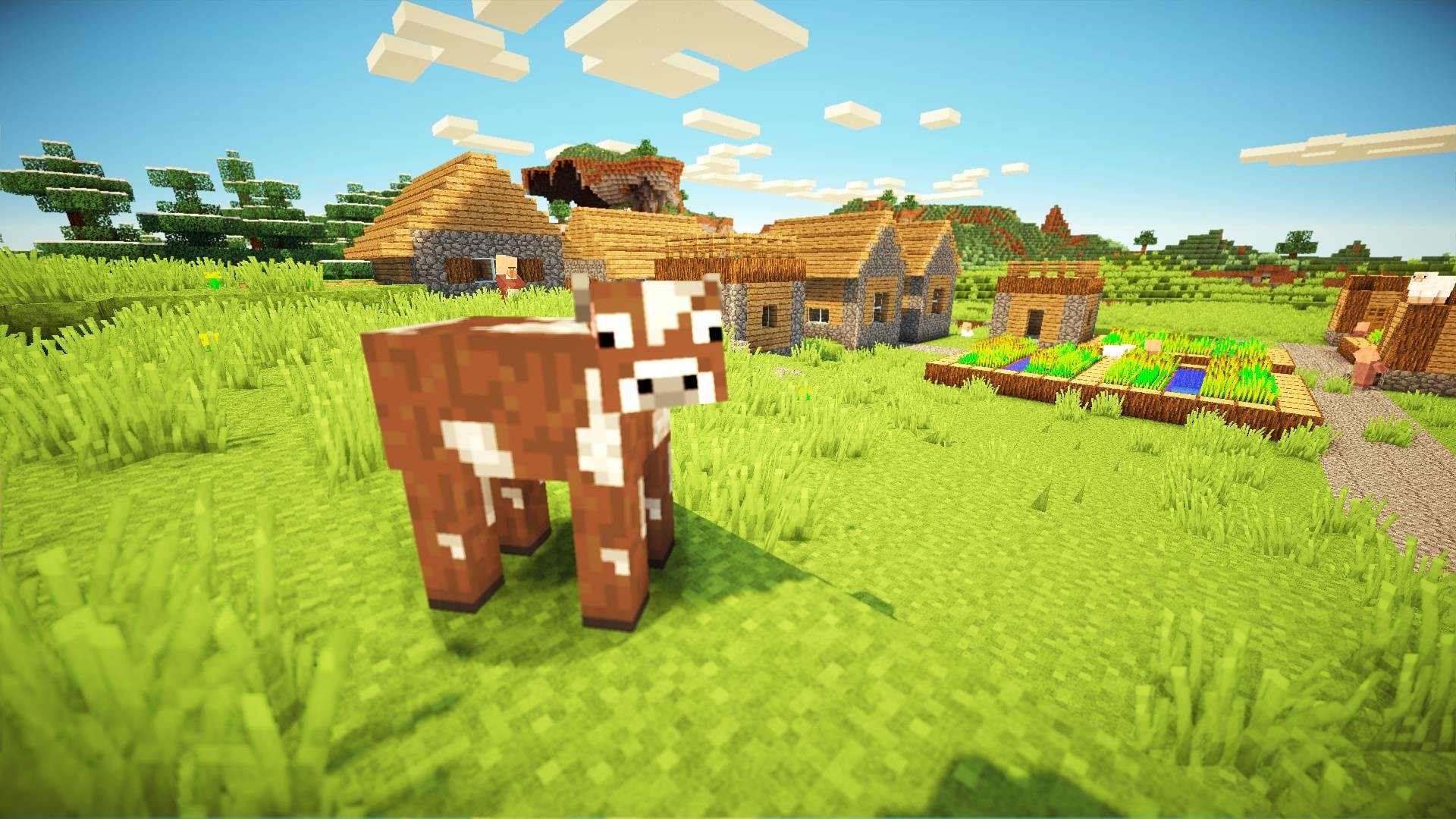The image appears to be a screenshot from the video game Minecraft, showcasing a vibrant, pixelated landscape. Dominating the center-left foreground is a brown and white blocky cow, complete with black square eyes and nostrils, typical of the game’s 8-bit art style. The cow stands amidst green grass. The background reveals a field dotted with six buildings, some complete with stone and straw structures shaped like traditional cabins, while others appear roofless or flat-topped. To the right of these buildings lies a small garden patch, likely for growing vegetables, and a pathway beside it where a character is visible. The scene also features rolling hills and blocky trees all rendered in Minecraft's signature blocky style. Above, the sky transitions from a darker shade at the corners to a light baby blue horizon, dotted with blocky clouds, adding to the quintessentially Minecraft aesthetic.